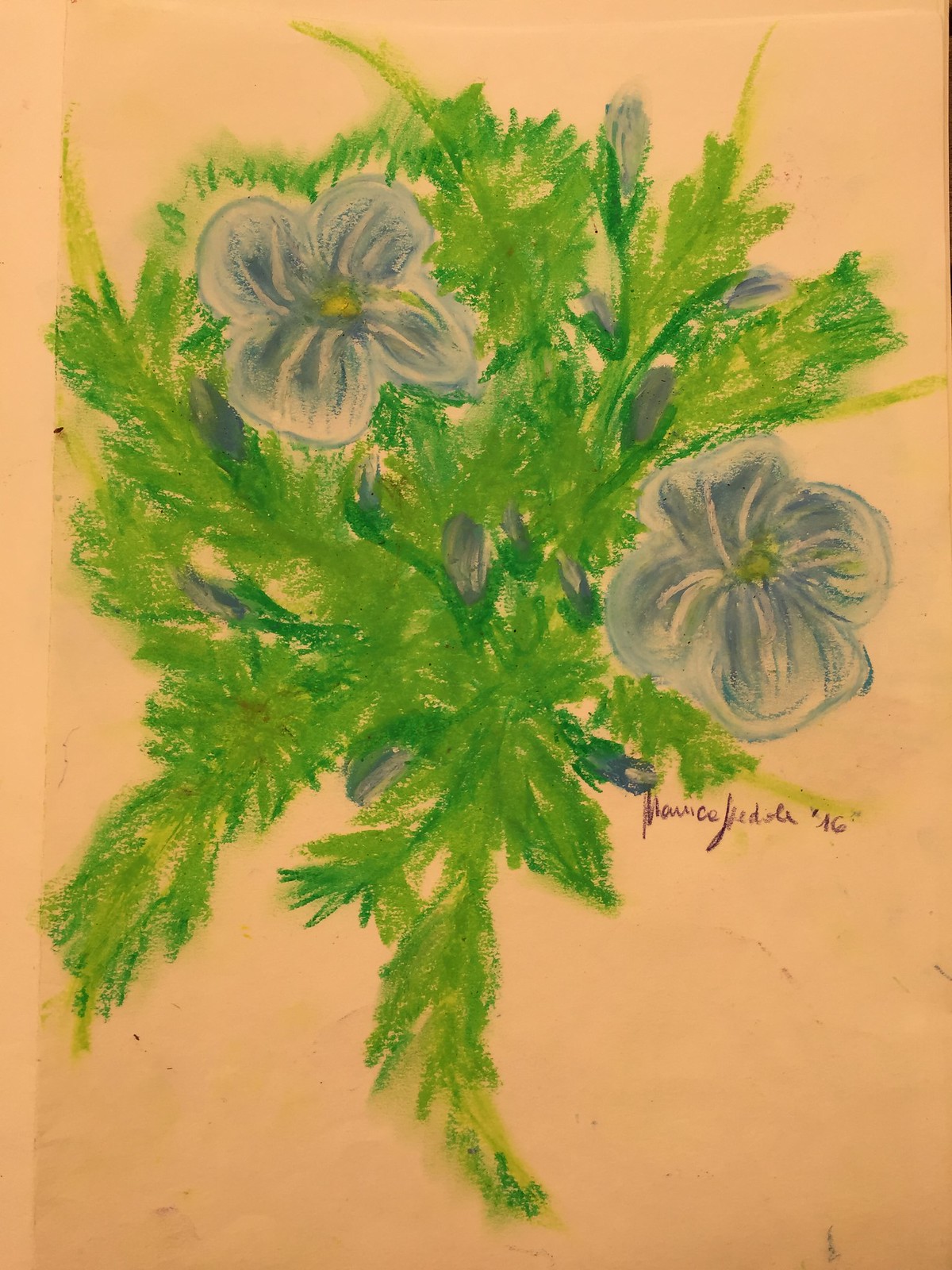This photograph captures an intricate drawing of a bouquet of flowers, created by an artist using either crayons, pastels, or chalk pencils. The central element of the artwork features a variety of purple pansies, showcasing shades that range from deep blue to vibrant purple with delicate highlights. The pansies are depicted in full bloom, framed by an abundance of lush green leaves, enhancing the composition's verdant appearance.

The drawing is rendered on a peach-colored background, which could be sketchbook paper or cardstock, providing a warm and subtle contrast to the vivid colors of the flowers and foliage. The artist's signature is distinctly marked in a rich burgundy hue at the bottom of the artwork. Additionally, the scene includes several flower buds in the background, suggesting growth and the promise of future blossoms, further adding depth and dimension to the piece.